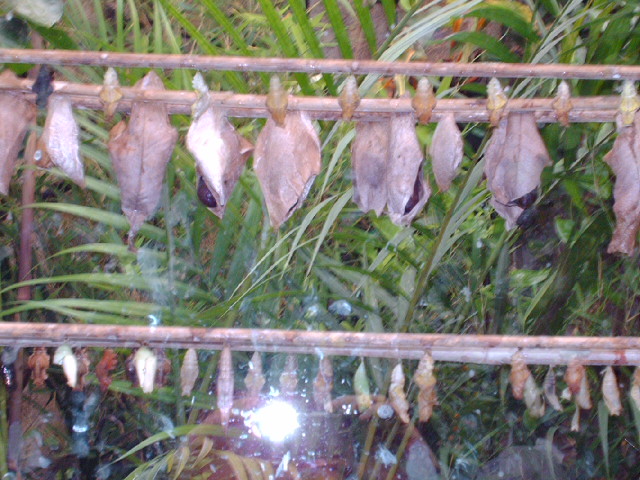The image appears to depict an outdoor zoo or science exhibit set amidst lush greenery and ferns, showcasing an enclosure dedicated to moths. Dominating the scene are two rows of wooden rods or bamboo sticks positioned horizontally and festooned with a fascinating array of objects. At the top, several large moths hang, possibly in a state of hibernation. Below them, ample cocoons of varying sizes and colors—gray, brown, and green—are attached, poised for the imminent emergence of moths or butterflies. The background is rich with verdant plant life, enhancing the naturalistic setting of the display. Additionally, a bright light emanates from the lower middle part of the image, which could be a flashlight or sunlight breaking through, although the exact source is indeterminate. The image is somewhat blurry, adding a sense of intrigue to the detailed and intricate exhibit.